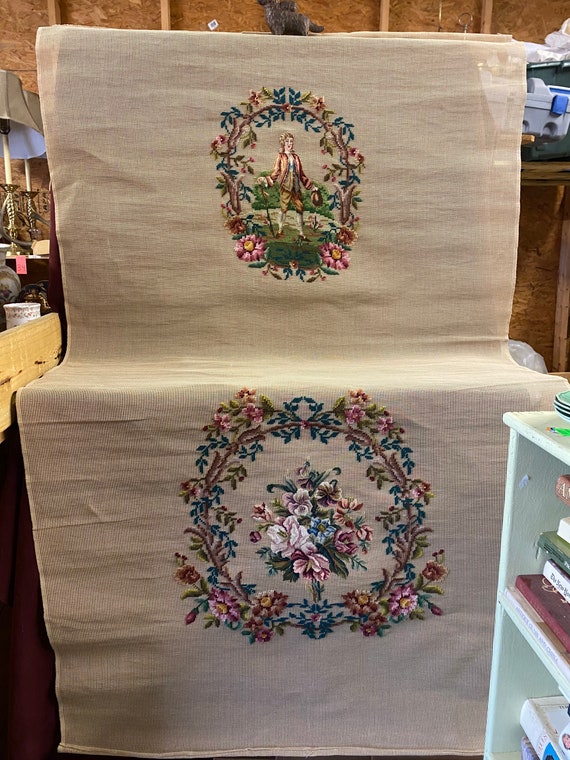The photograph showcases an intricately stitched tapestry or long piece of fabric positioned almost vertically from top to bottom. It appears to be placed indoors, possibly in a rustic setting with rough, wooden walls that resemble plywood. The tapestry is draped over a flat horizontal surface akin to a table or bench, creating a sense of depth and texture in the image. The fabric itself is light-colored, possibly off-white or cream, and features detailed designs. 

At the top portion of the tapestry, there is an oval border adorned with leafy, flowery patterns, depicting a historical figure. The man, dressed in old-fashioned attire including knickers, high socks, a frocked jacket, and a vest, stands holding a hat in one hand and a cane in the other. His presence is juxtaposed against a backdrop of green grass, suggesting a pastoral scene.

Further down the tapestry, another larger circular design mirrors the flowery, leafy, and viney motifs. Inside this border is a vivid bouquet comprising blue, pink, and red flowers, accompanied by green leaves, exhibiting the tapestry's elaborate needlework. 

To the right of the tapestry, a shelf filled sparingly with books and topped with plate-like objects is visible, adding to the room's quaint charm. On the left, there's a lamp with a lampshade, contributing to the warm, indoor ambiance. The photo is taken from a standing position, centrally focusing on the tapestry, emphasizing its detailed artistry and the colors which include pink, blue, light mint green, brown, tan, and off-white.